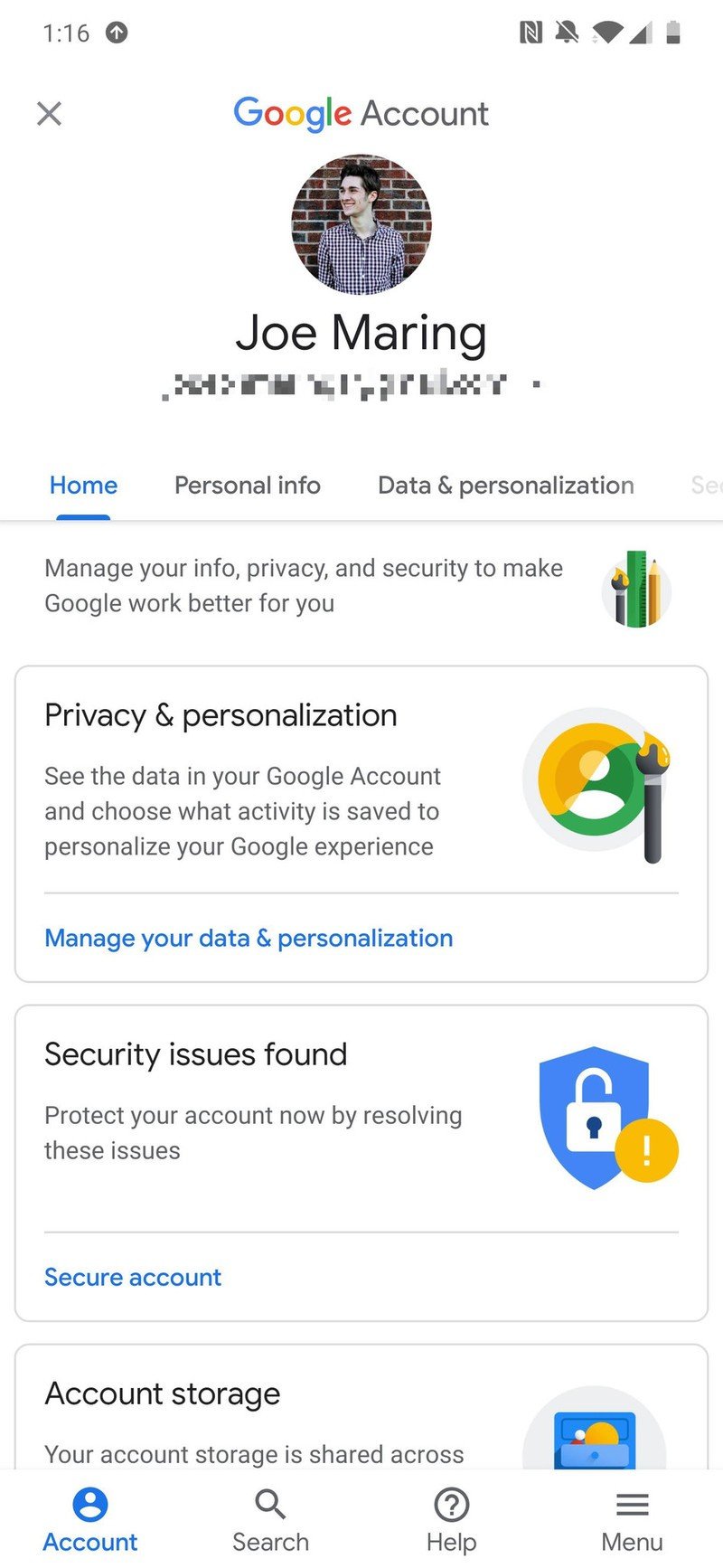Screenshot Description: Joe Maring's Google Account Management Page

The image is a detailed screenshot of Joe Maring's Google account management page. The header prominently displays the name "Joe Maring" with his last name spelled "M-A-R-I-N-G." Some adjacent text appears pixelated and unreadable. Below the header, there are several navigational tabs: "Home," "Personal info," "Data & personalization," "Manager info," "Privacy & security," each aimed at helping Joe manage various aspects of his Google account.

On the main portion of the page, a white box titled "Privacy & Personalization" is visible, offering Joe options to see the data in his Google account and choose what activity should be saved to personalize his Google experience. The box includes a prompt to "Manage your data and personalization."

Another prominent feature is a "Security Issues Found" box, which alerts Joe to potential security problems with his account and provides an option to "Secure account" by resolving these issues.

Additionally, there is a section labeled "Account Storage," indicating that Joe's account storage is shared across various services. To find out the specific details of this shared storage, Joe would need to click on the provided link or option.

The screenshot also reveals several options in a menu-like format, including "Account," "Search," "Help," and "Menu," providing Joe with easy access to different functionalities within his account.

Overall, this Google account management page snapshot allows Joe Maring to navigate, personalize, and secure his account effectively, featuring multiple tabs and sections dedicated to various aspects of account management.